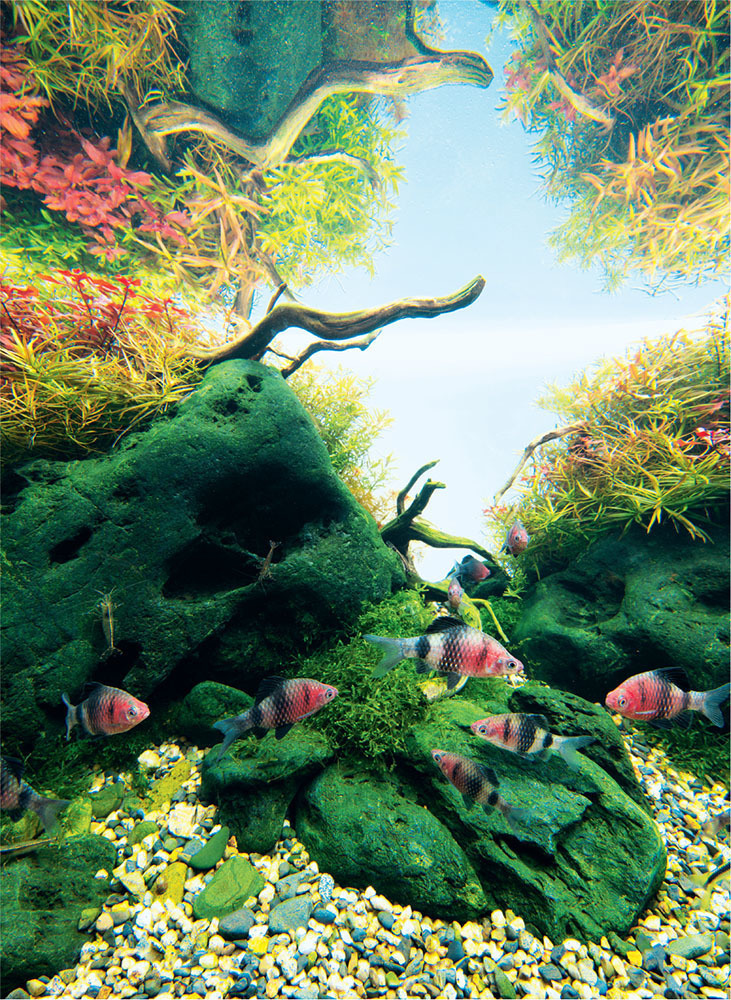The image depicts a vibrant underwater scene that appears to be a detailed artwork or a digitally altered photo. At the bottom, a layer of small, gray, white, and yellow aquarium-style rocks creates the foundation. Rising from these rocks are green, knobby formations, which could either be larger rocks or undersea mountains. Interspersed amongst these formations, there are patches of yellow and green grass-like shoots and thick aquatic branches extending outward.

A school of fish, numbering six or seven, swims gracefully in the foreground. These fish have striking red and black striped bodies, adding a lively contrast to the scene. The underwater setting is complemented by additional red flowers located in the upper left corner, contributing to the vivid color palette of the image.

The upper part of the image showcases a clear blue expanse, which at first glance resembles the sky but is actually a depiction of the pristine water above. This clear area enhances the fantastical feel of the artwork, making it appear almost as if the scene is taking place in a surreal aquarium setting, perhaps in someone’s living room or bedroom. The overall composition exudes a sense of tranquility and beauty, blending realistic and fantastical elements seamlessly.